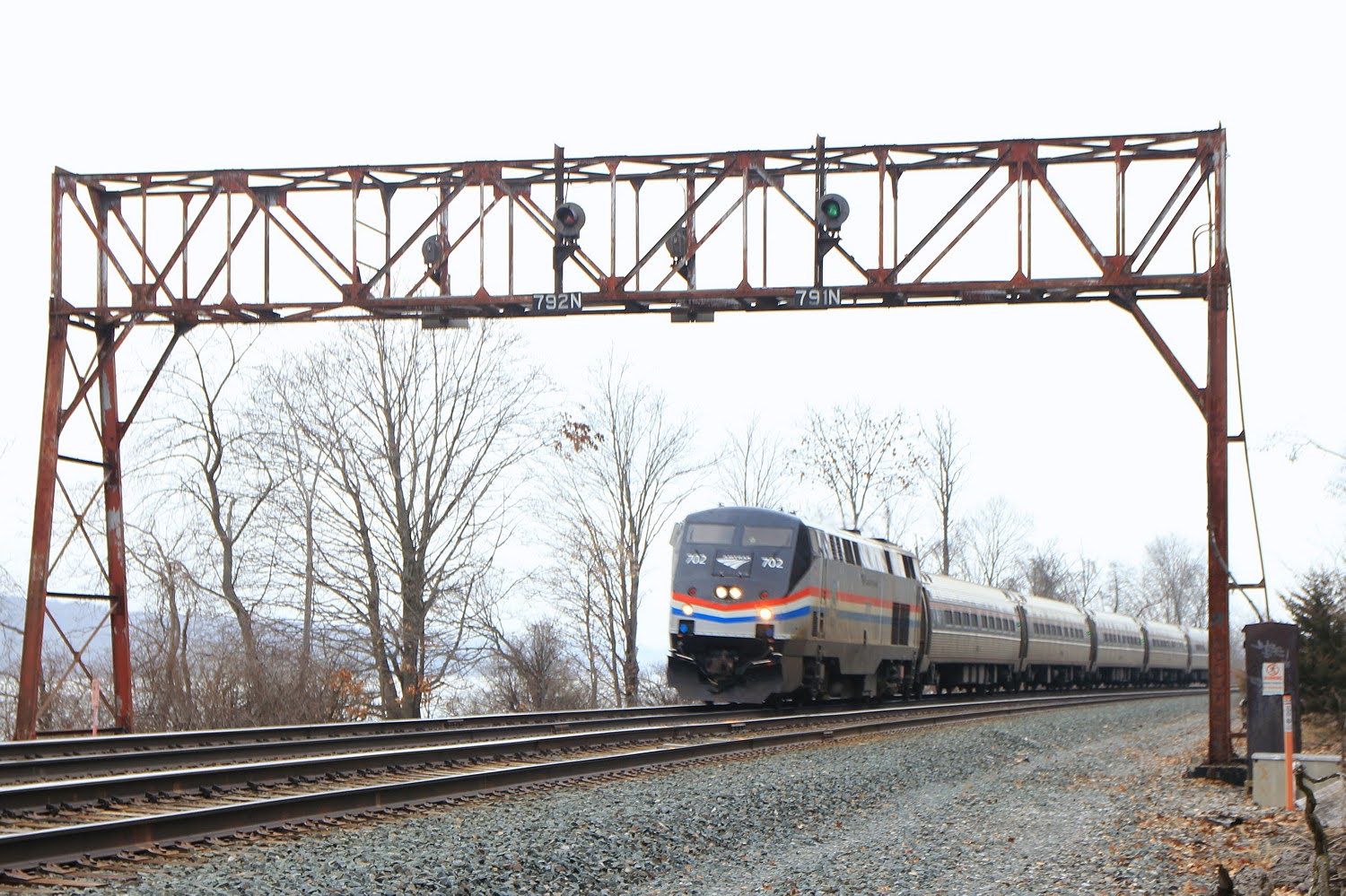In this photograph, a standard Amtrak train, identifiable by its red, white, and blue ornamentation adorning the front engine and sides, is captured traveling on the rails through a wooded area. The train, featuring the number 702, consists of seven visible cars. The trees in the background are devoid of leaves, suggesting it is either fall or winter, and the sky is overcast, creating a white backdrop. The train is seen approaching a large metal scaffolding, which appears to function as a light switch station. To the left of the train, there is a noticeable drop-off leading down to a likely river, with hills and mountains visible on the opposite side. The ground alongside the track is covered in gray gravel and rocks.